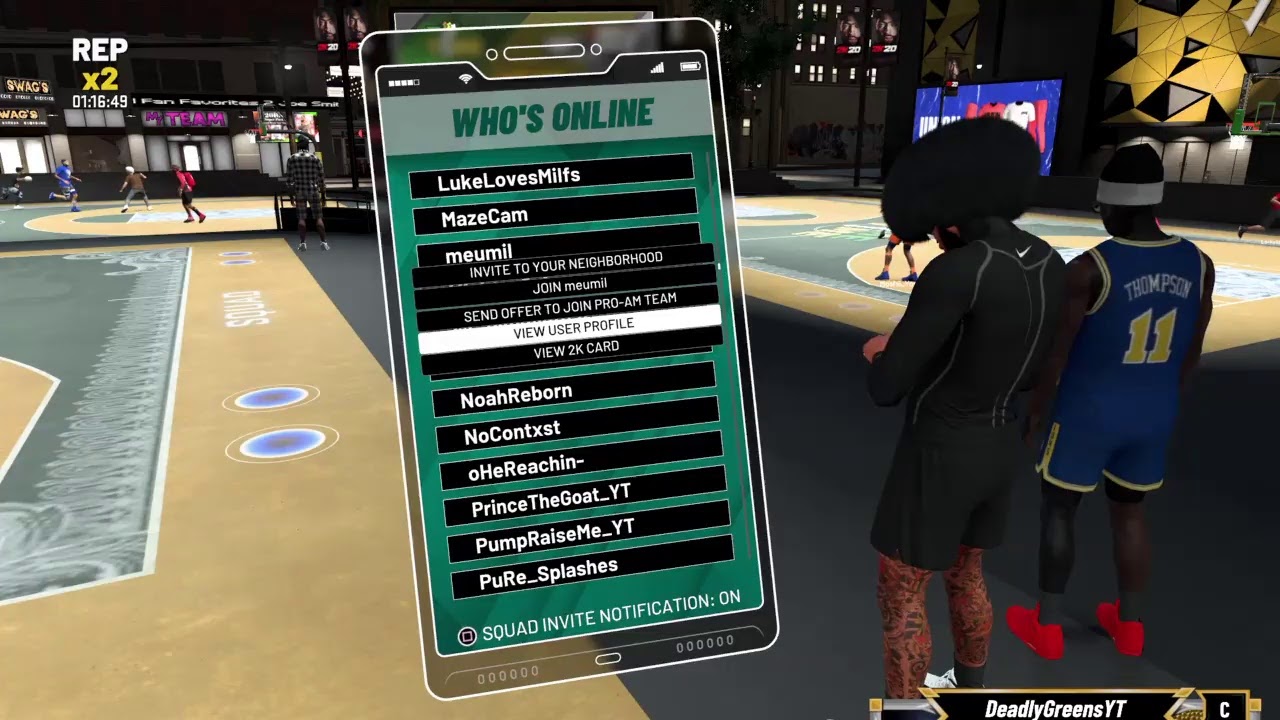In this horizontally rectangular image, captured from a video game, a bustling outdoor gaming environment is depicted, featuring various courts in the background, such as basketball courts. On the right side of the frame stand two players facing away from us. The player to the extreme right is dressed in a blue tank top with yellow borders, reminiscent of a basketball jersey, emblazoned with the name "Thompson" and the number 11 on the back. This athlete, in addition to their uniform, is wearing shorts that reveal fully tattooed legs. Standing next to him, slightly to the left, is another player garbed entirely in black, including a long-sleeve top. Both players are wearing shorts. Overlapping the figures on the left is an in-game cell phone display, detailing the online status of various players. At the bottom of this overlay, a squad invite notification is visible, highlighting the social interactions within the gaming environment.